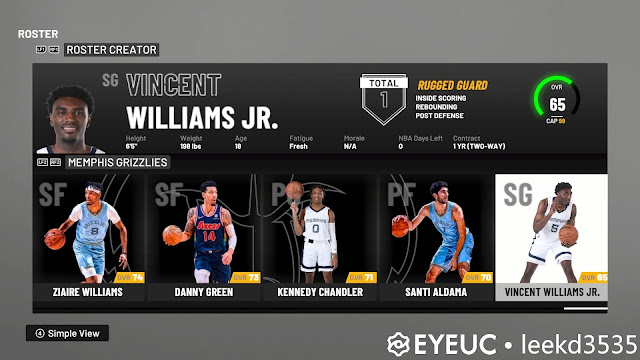This image depicts the roster for a basketball team, presented on a gray background. The word "ROSTER" is prominently displayed in white font in the upper left-hand corner. Below this, the term "Roster Creator" is written, also in white, on a dark gray background strip. 

Centrally, there is an embedded section within the image showing detailed information about a specific player. This section features a small picture of the player's head and upper shoulders to the left, with "SG" (indicating the position Shooting Guard) marked in the top left corner of this smaller image. The player's name, "Vincent Williams Jr.," is prominently displayed to the right of the image. Further to the right is a small flag icon followed by the word "TOTAL" and the number "1."

The player’s profile notes key skills and attributes: interior scoring, rebounding, and post defense, making him a versatile and valuable player on the team. The comprehensive layout provides a clear and informative overview of the player and the construction of the roster.